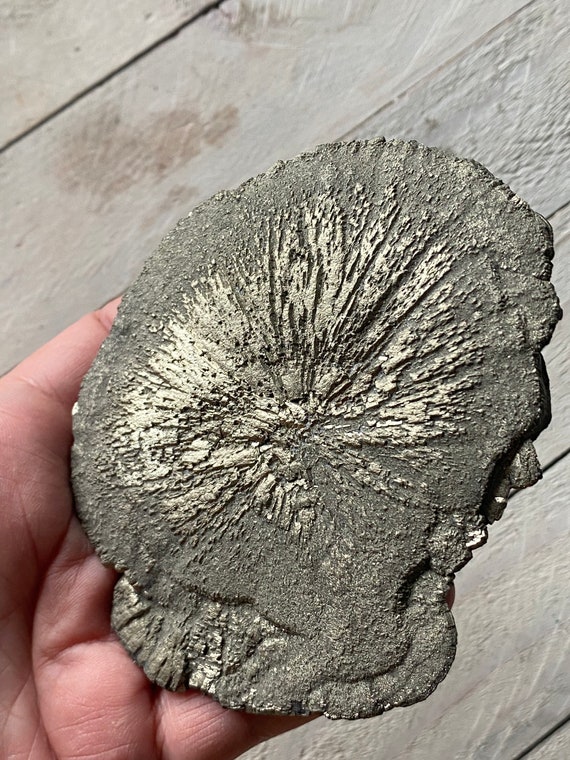This close-up, overhead photograph captures a fossil held in the palm of a person with light skin. The white-painted wooden floor provides a subdued background that accentuates the fossil's details. The rugged, flat fossil, encased in dirt and shaped almost like a flattened circle with jagged edges, is primarily gray. It features a striking, lighter gray pattern that resembles radiating lines from a central point, akin to the sun's rays. This intricate texture suggests the fossil may be from a sea creature, with parts of its shell creating the detailed impressions. In the image, parts of the person's palm, pinky, and thumb are visible at the edges, focusing attention on the fascinating fossil cradled gently in their hand.